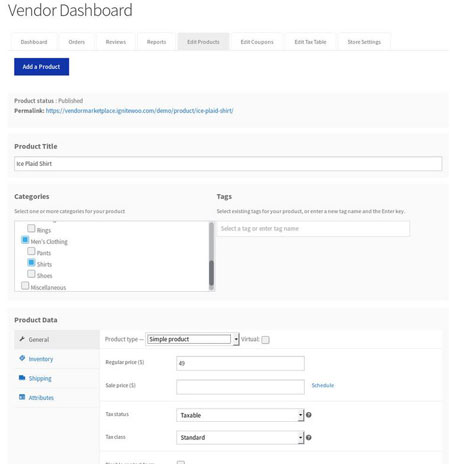The image displays a vendor dashboard against a clean, white background. At the top of the dashboard, there are multiple rectangular tabs labeled: Dashboard, Orders, Receipts, Reports, Edit Products, Edit Coupons, Edit Text Table, and Store Settings. A prominent blue rectangle features options such as Add a Product, Production, Published, and Permalink. A website address is also displayed in blue, alongside a section for the product title.

Within the main content area, there is a detailed form for adding or editing a product, illustrated with an example of a "Plaid Shirt" or "Ice Plaid Shirt." The form includes multiple categories with checkboxes, where "Men's Clothing" and "Shirts" are selected, while others like "Rings," "Pants," "Shoes," and "Miscellaneous" remain unchecked. Tags can be added in a designated box by selecting from existing ones or entering new tag names.

Further sections of the form are organized under tabs labeled Product Data, which include General, Inventory, Shipping, Airtime, and Attributes. The General tab is the active section, indicated with black text, while the other tabs are displayed in blue. The dashboard is packed with numerous fields and options to comprehensively manage and configure product details.